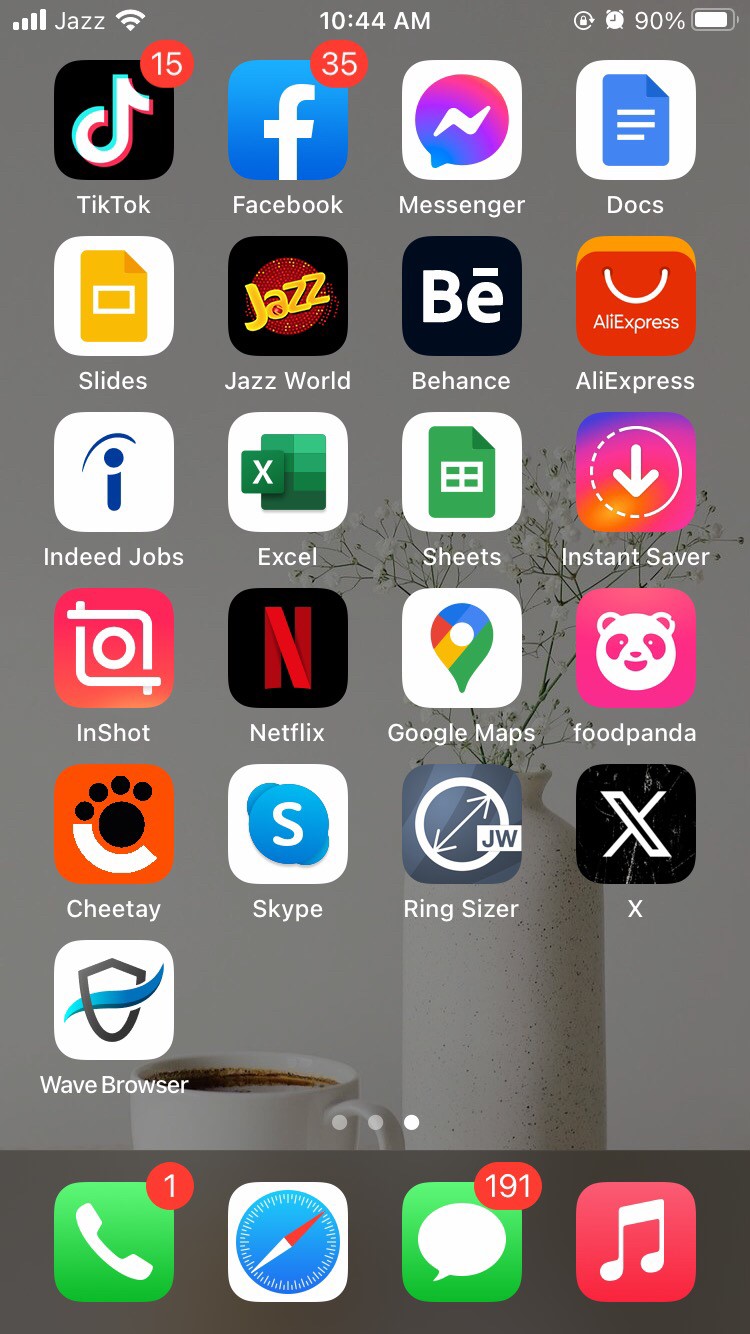This screenshot captures a secondary screen on an Apple iOS mobile device. At the top, there is a status bar displaying, on the left, cell phone signal and quality icons. Centrally positioned is the current time, shown as 10:44 a.m., and on the right, a battery icon indicating 90% charge alongside an alarm clock icon.

The screen features a rich array of 21 application icons. In the top-left corner is the TikTok app, marked with a notification badge displaying '15'. Adjacent to it is the Facebook app, distinguished by a red notification badge with '35'. The last icon on this page, positioned at the bottom-right corner, is the Wave browser, identifiable by its white background and a shield containing a blue wave.

The navigation bar at the bottom of the screen includes four icons: a talk button, a compass button, a messages button with a high notification count of '191', and a music button. The background image for this screen showcases a jar and a cup of coffee, lending a cozy atmosphere to the user interface.